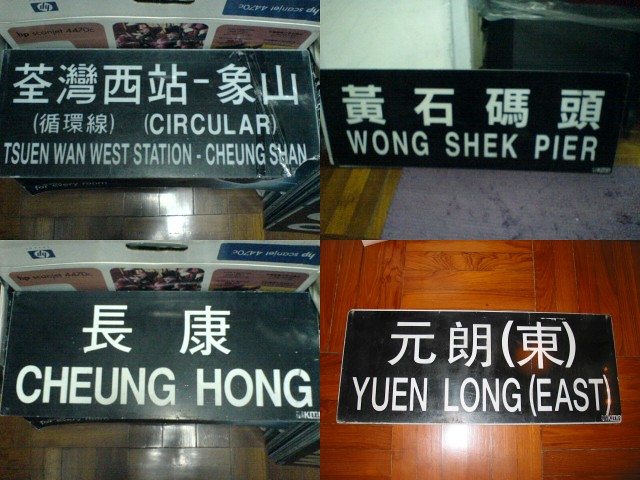This image is a collage consisting of four distinct photos, each showcasing a different black sign with white lettering, bearing both Asian characters and English translations. The upper left sign, labeled "Tsuyinwan West Station, Changshan," features a row of Asian characters and rests against a box, likely in someone's home. The upper right sign, marked "Wong Shik Pier," is situated on a carpeted floor, leaning against a white post. The lower left sign, which reads "Cheung Hong Below," is balanced against a similar box, sharing the same setup as the upper left sign. The bottom right sign, stating "Yuen Long East Below," lies atop a polished brown wooden floor, distinctively brighter than the other backgrounds. Each sign appears to be photographed in different settings, emphasizing the varied home environments in which they currently reside rather than being installed in their intended locations.